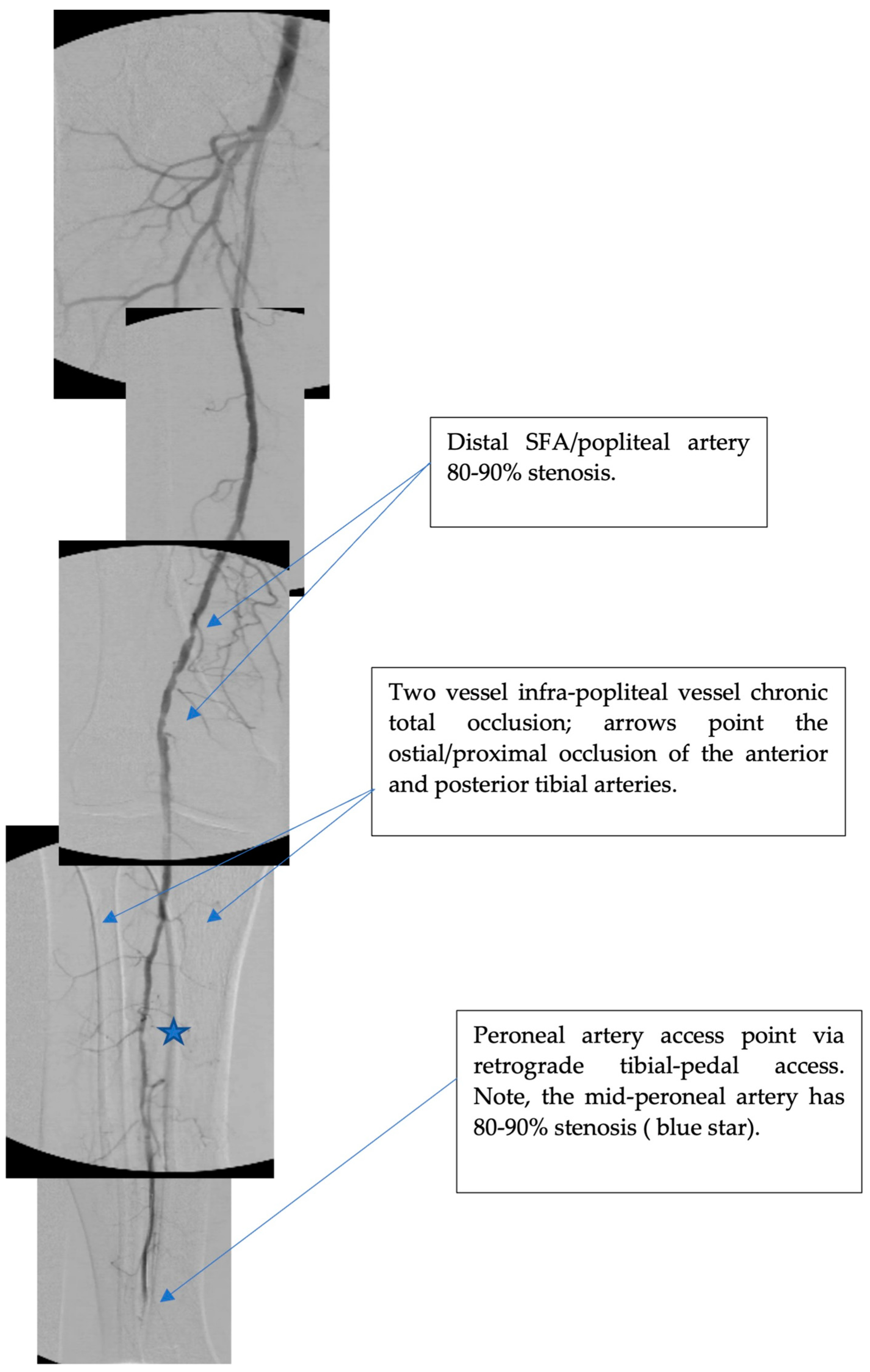The image in question is a detailed scientific diagram showcasing a person's artery, composed of multiple smaller images stitched together to present a continuous view of the artery. This methodology seems necessary as the artery is exceptionally long and thin, resembling a tree root, making it difficult to capture in a single shot. The artery is visualized in shades of gray and black against a whitish-gray backdrop, indicative of medical imaging techniques.

On the right side of the diagram, various text boxes with thin black borders filled with black Roman text provide important annotations. These annotations are accompanied by blue arrows and stars pointing to specific sections of the artery. Notable labels include "two-vessel infraportable vessel chronic total occlusion" and "distal SFA artery 80-90% stenosis," with arrows indicating the osteo-proximal occlusion of the anterior and posterior tibial arteries. The image also highlights regions of the peroneal artery, indicating an access point via retrograde tibial fetal access and mentioning another 80-90% stenosis in the mid-peroneal artery marked by the blue stars.

Overall, the diagram appears to be a comprehensive presentation of arterial conditions, likely utilized for medical analysis or diagnostic purposes, emphasizing areas of significant stenosis and occlusion.